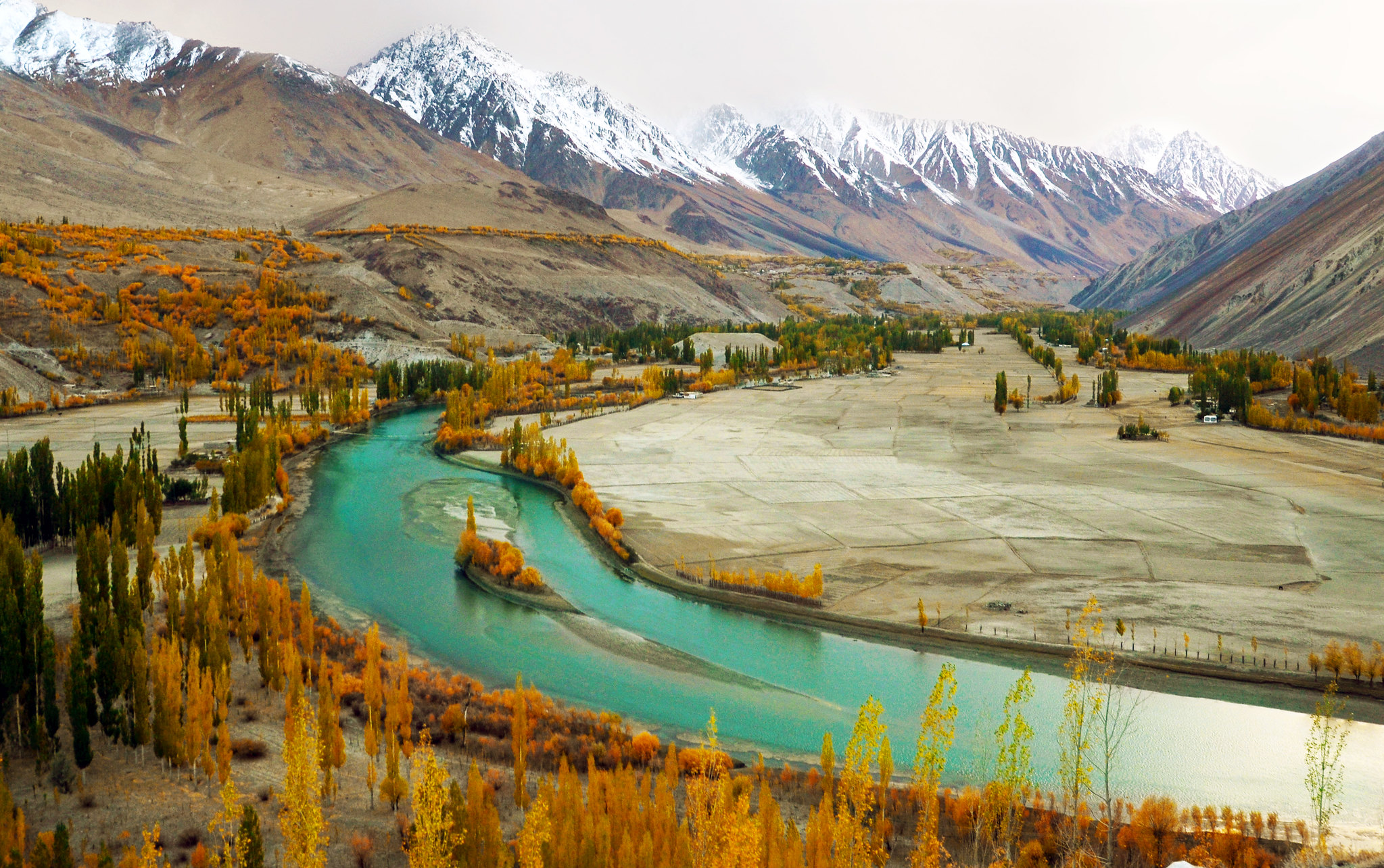This is a detailed, picturesque painting capturing a serene daytime mountain landscape in winter. The scene features majestic snow-capped mountains transitioning into rugged, earthy terrain as they descend. A diverse array of trees, predominantly brown, populates the landscape—ranging from tall, slender trunks to shorter, bushier forms. A grey concrete walkway winds along the mountain's edge, bordered by more trees. 

In the foreground, new green and brown growth hints at the rebirth amidst the colder season. A tranquil body of water runs through the scene, featuring a pointy boat laden with brown trees, moving downstream. To the left, there is a sparse cluster of green trees. The painting also subtly reveals two indistinct figures in the distance, adding a touch of mystery to the serene, wintry tableau.